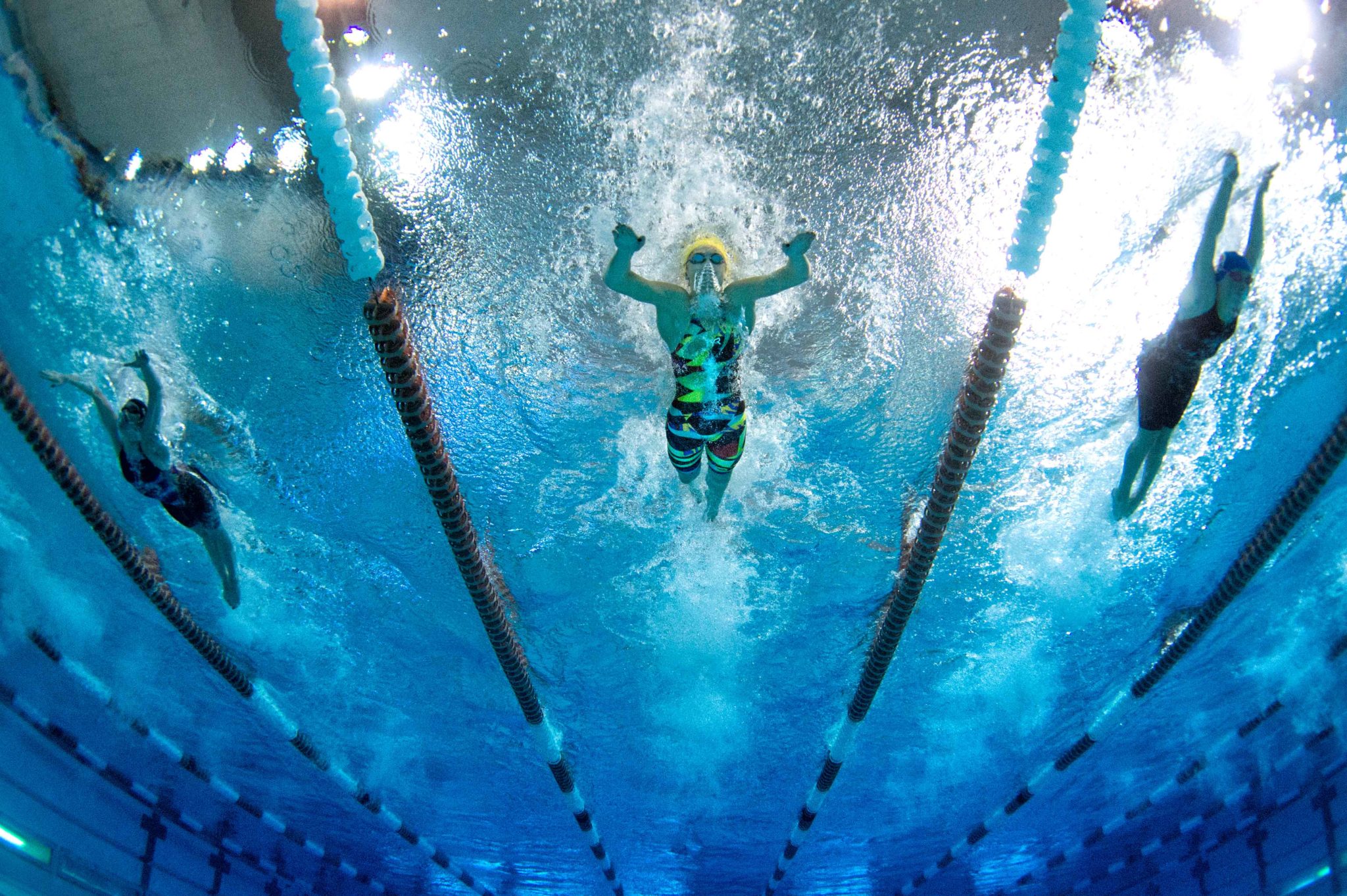An underwater view captures three competitive swimmers in their lanes, marked by red and white doughnut-shaped dividers, in an Olympic-sized pool. The backdrop reveals a white ceiling with visible lights, casting shimmering silver reflections through the varying shades of blue water, ranging from light to midnight blue. Centered is a male swimmer in a multicolored swimsuit and yellow swim cap, the focal point of the image, seemingly performing a breaststroke with bent elbows. Flanking him are two female swimmers. On the left, a woman in a black swimsuit with floral patterns appears to have just completed a turn, indicated by her body structure and form. On the right, another woman, also in a black swimsuit but with a blue swim cap, looks poised to make her turn. The photograph, taken from the pool's floor looking upward, captures the trail of bubbles from their breathing and the dynamic motions of their strokes, emphasizing the intense competition and fluidity of the scene.